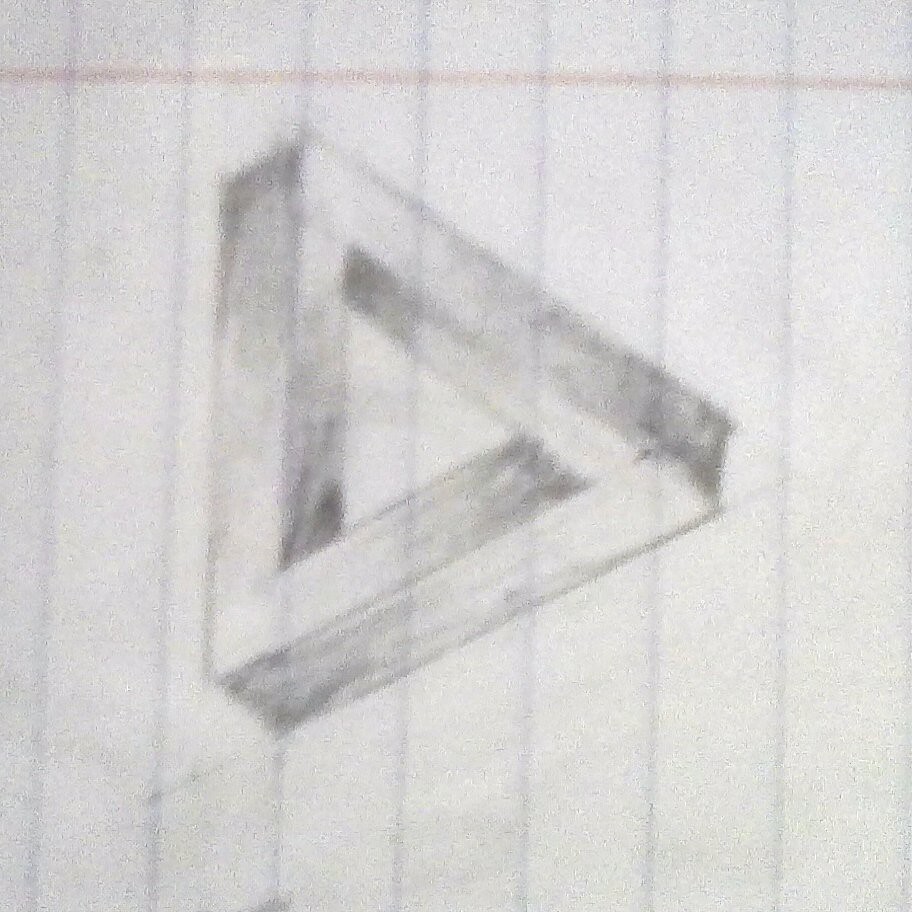This image features a very blurry photograph of a pencil sketch drawn on a piece of standard lined paper, the type typically used by students in school. The paper is oriented sideways, showcasing light blue horizontal lines running across it with a single pink line running perpendicularly at the top, intersecting with all the blue lines. The sketch itself appears to be slightly smudged, enhancing the hand-drawn quality of the piece. It depicts an optical illusion involving an impossible geometric shape—specifically, a three-dimensional triangle where each side connects to the next in a manner that defies logical spatial arrangement. The shading in the drawing effectively creates a three-dimensional effect, further emphasizing the illusion.